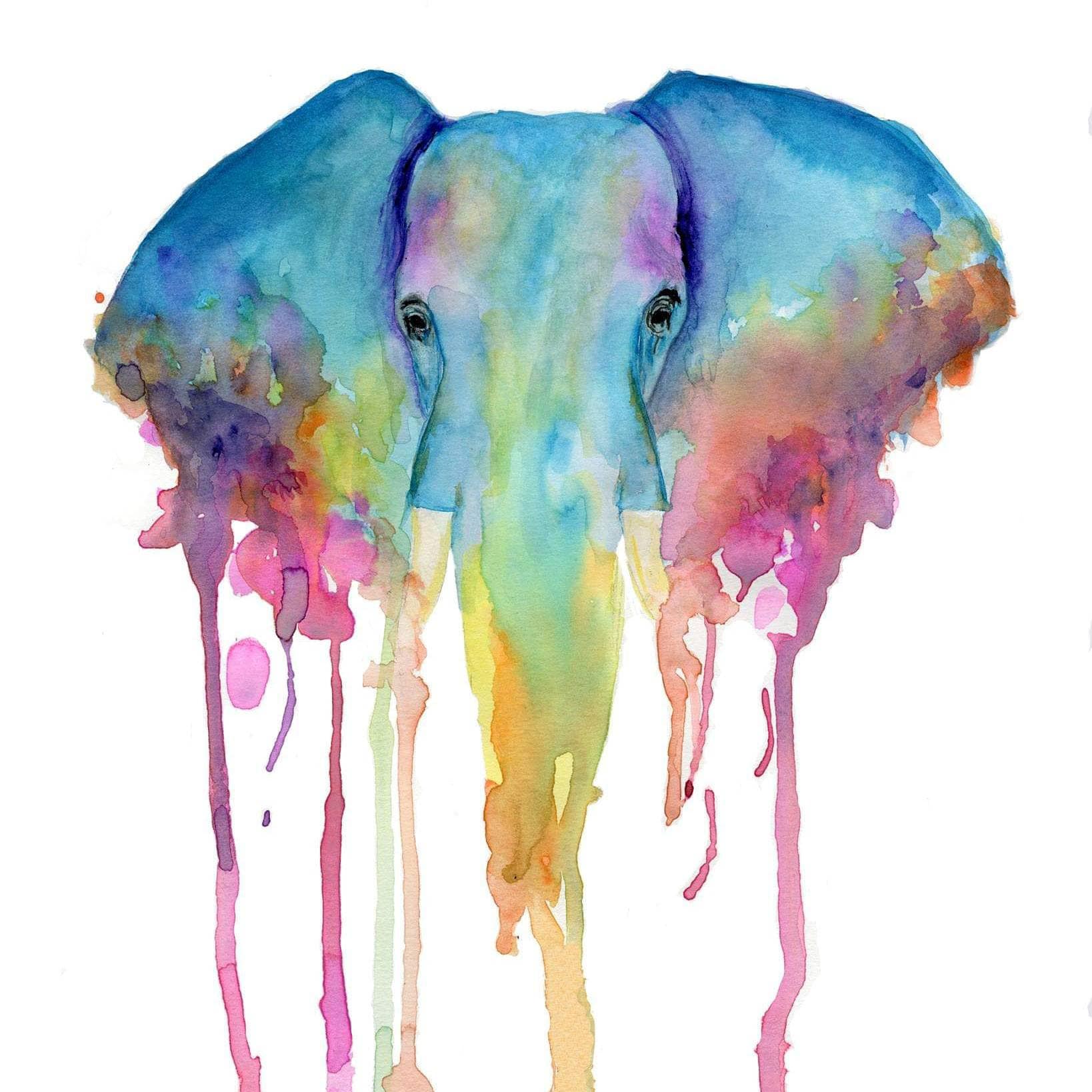This image is a digital watercolor rendering of an elephant, showcasing a blend of artistry and fluid motion. It primarily features the elephant's head, with expressive black eyes and visible tusks. The elephant's head and ears are rendered in light grays, blues, and whites, conveying a serene and ethereal quality. The ears are painted in blue with vibrant edges that transition into splashes of pink, purple, green, yellow, and orange. Complementing this, the trunk starts whole but quickly dissolves into streaks of dripping paint, mimicking the fluidity of traditional watercolor as it extends to the bottom of the image. The entire composition is set against a stark white background, giving the impression of the elephant being suspended mid-air, with paint flowing freely off its form, blending symbolism with abstract aesthetics.